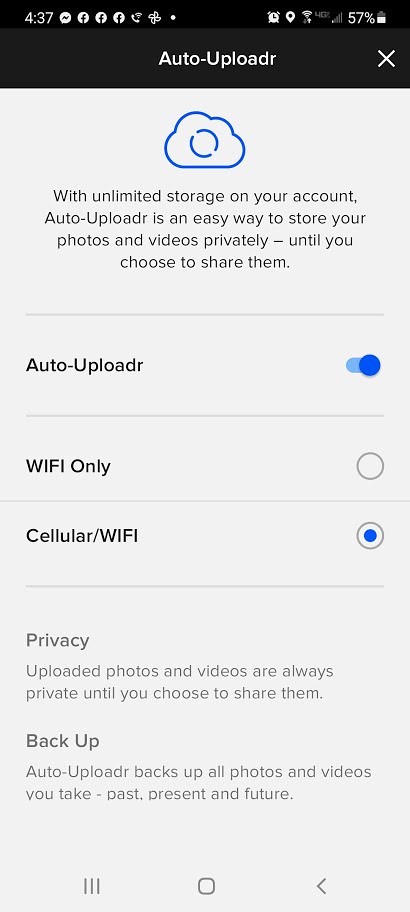This is a detailed image caption for a phone screenshot:

---

The screenshot, taken from a smartphone, shows the display at 4:37 PM. At the top of the screen, various icons are visible: notifications for Facebook Messenger and Facebook, along with symbols representing an alarm clock, location services, Wi-Fi signal, cellular signal bars, and the battery level, which is at 57%. 

The URL bar reads "auto-uploader." Below, a blue cloud graphic is displayed with the following text: "With unlimited storage on your account, auto-uploader is an easy way to store your photos and videos privately until you choose to share them."

On the left side of the screen, the text "auto-uploader" is written. On the right side, there is a toggle switch, currently enabled and highlighted in blue. Below this, the text "Wi-Fi only" is accompanied by an unchecked circular check mark. Beneath it, "Cellular/Wi-Fi" shows a similar circular check mark that is checked.

Further down, the word "privacy" is bolded, followed by the explanation that "Uploaded photos and videos are always private until you choose to share them." The next section, "backup," details that the "Auto-uploader backs up all photos and videos you take, past, present, and future."

At the bottom of the screen are three navigation icons: three horizontal lines on the left, a square in the middle, and a left-pointing arrow on the right.